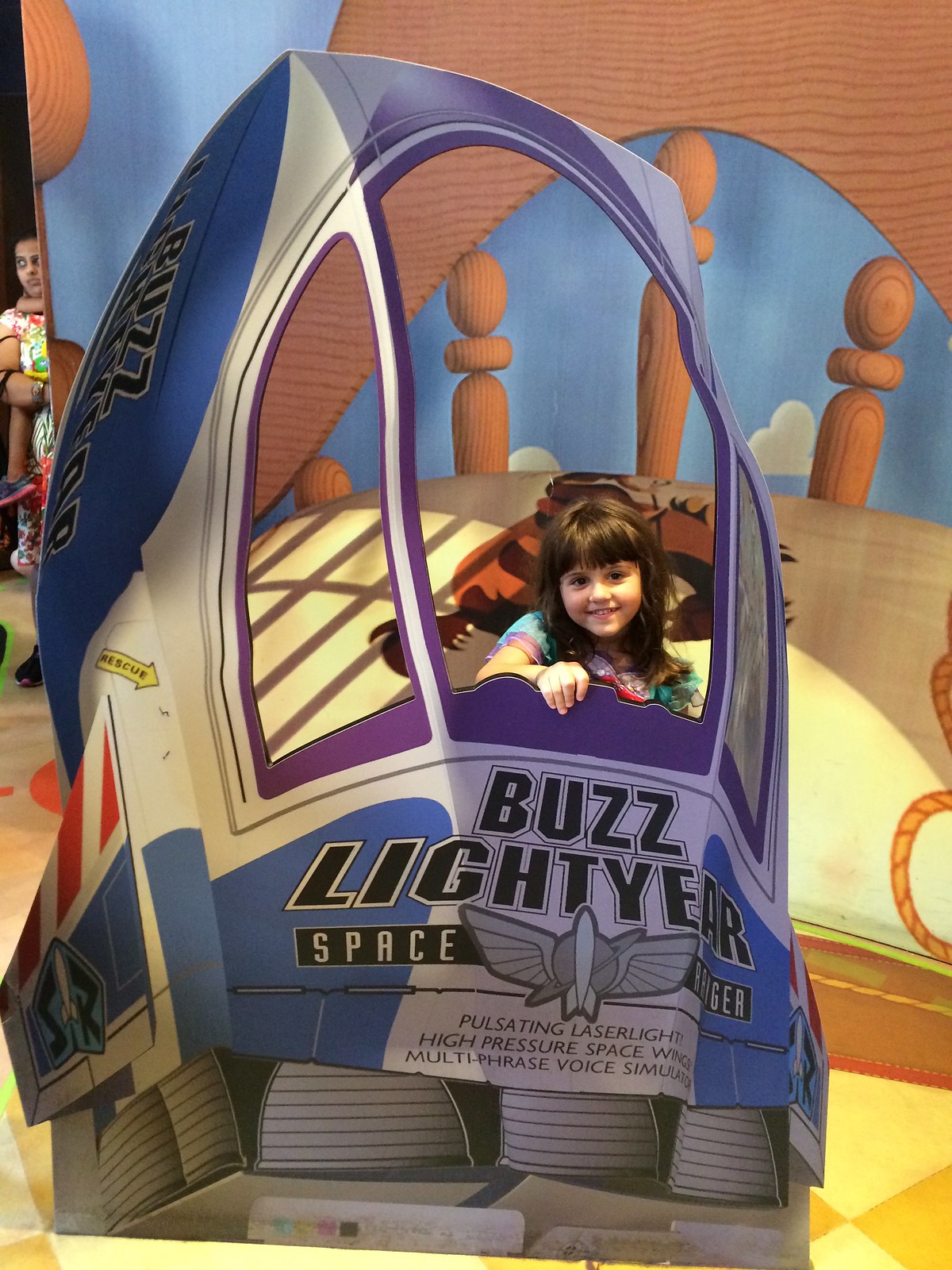The image is a vertically-oriented indoor photograph capturing an enchanting scene inspired by Disney's Toy Story. At its center stands a young girl, approximately six or seven years old, likely of Caucasian descent, who is smiling brightly at the camera. She has shoulder-length straight brown hair with bangs, and she is dressed in a multi-colored top. Her right hand is posed on the open window of a meticulously crafted stage prop: a cardboard spaceship designed to resemble Buzz Lightyear’s iconic space ranger box.

The Buzz Lightyear spaceship is predominantly white with purple accents around the cockpit area, and features blue elements on the side. Prominently, the name "Buzz Lightyear" is inscribed in black both on the side and the front of the spaceship. Beneath it, the words "Space Ranger" appear alongside an emblem depicting Saturn with a rocket and wings. Additional text on the spaceship reads: "Pulsating Laser Lights," "High-Pressure Space Wings," and "Multi-Phase Voice Simulator."

The backdrop emulates Andy's room from Toy Story, showcasing a sky-blue wall adorned with clouds and featuring Andy’s bed. Notable details include a large pillow with an illustration of Woody riding Bullseye, enhancing the nostalgic atmosphere. In the upper left-hand corner of the image, a red rope indicates an organized queue, with more people awaiting their turn to pose with the spacecraft. The floor beneath the scene is patterned in a cheerful yellow and orange checkered design, adding to the vibrant and playful ambiance of the photograph.